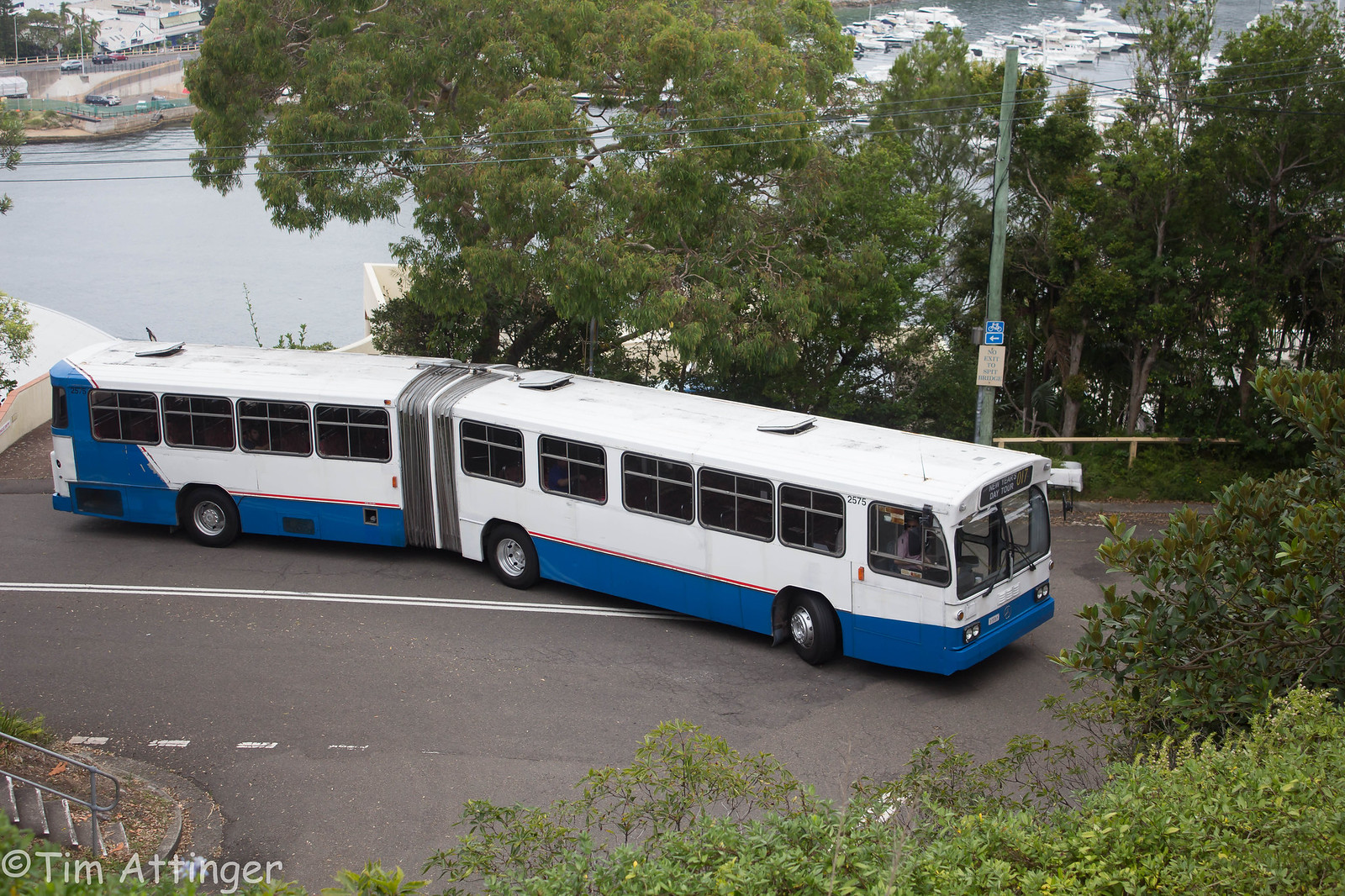The image depicts a bird’s-eye view of a street scene featuring a long, articulated bus, commonly known as an accordion bus, navigating a turn. The bus is distinctive with its white top and midsection, contrasted by a solid blue lower half. It showcases black tires and white dividers on the black road. The background is rich with greenery, including numerous trees and bushes, partially obstructing the view of a large, calm body of water behind them. White boats are docked by the waterfront, hinting at a serene harbor scene. The bus bears the marking "Tim Attinger" in white lettering, contributing to its unique identification.